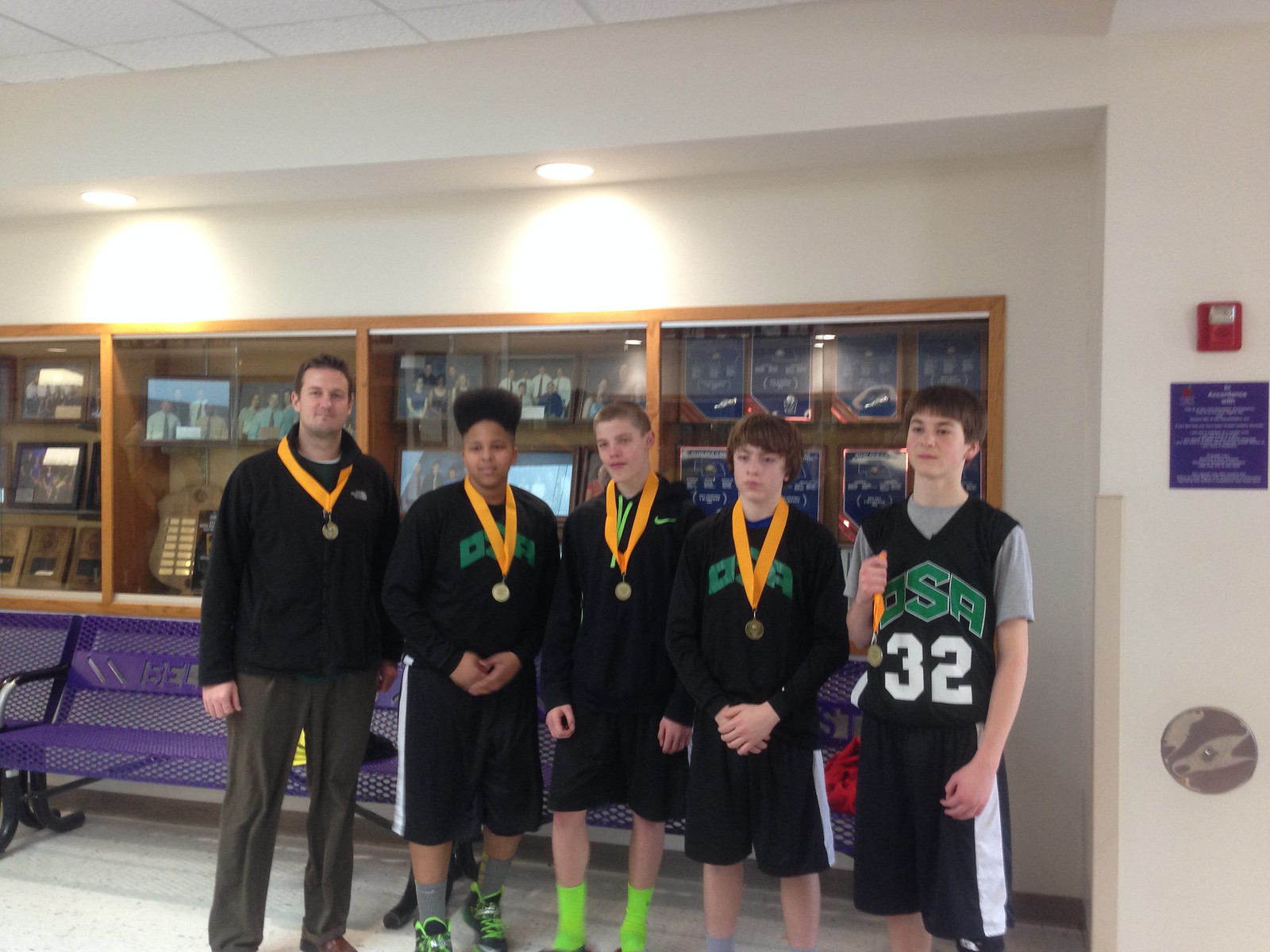The image depicts a group of five young men, predominantly teenagers, standing side by side proudly displaying yellow medals around their necks. They are dressed in matching black and white uniforms, with "USA" or "O.S.A." emblazoned on their shirts, and their shorts feature white stripes down the sides. The setting appears to be indoors, possibly in a room or corridor with white walls, blue benches, and display cases containing pictures and possibly other awards or trophies. A purple item is hanging on the wall. Positioned to the left is an older man, likely their coach, who stands out by wearing pants instead of shorts. One of the young men holds his medal in his hand while the others wear theirs around their necks. Despite their achievements, their expressions appear rather subdued.